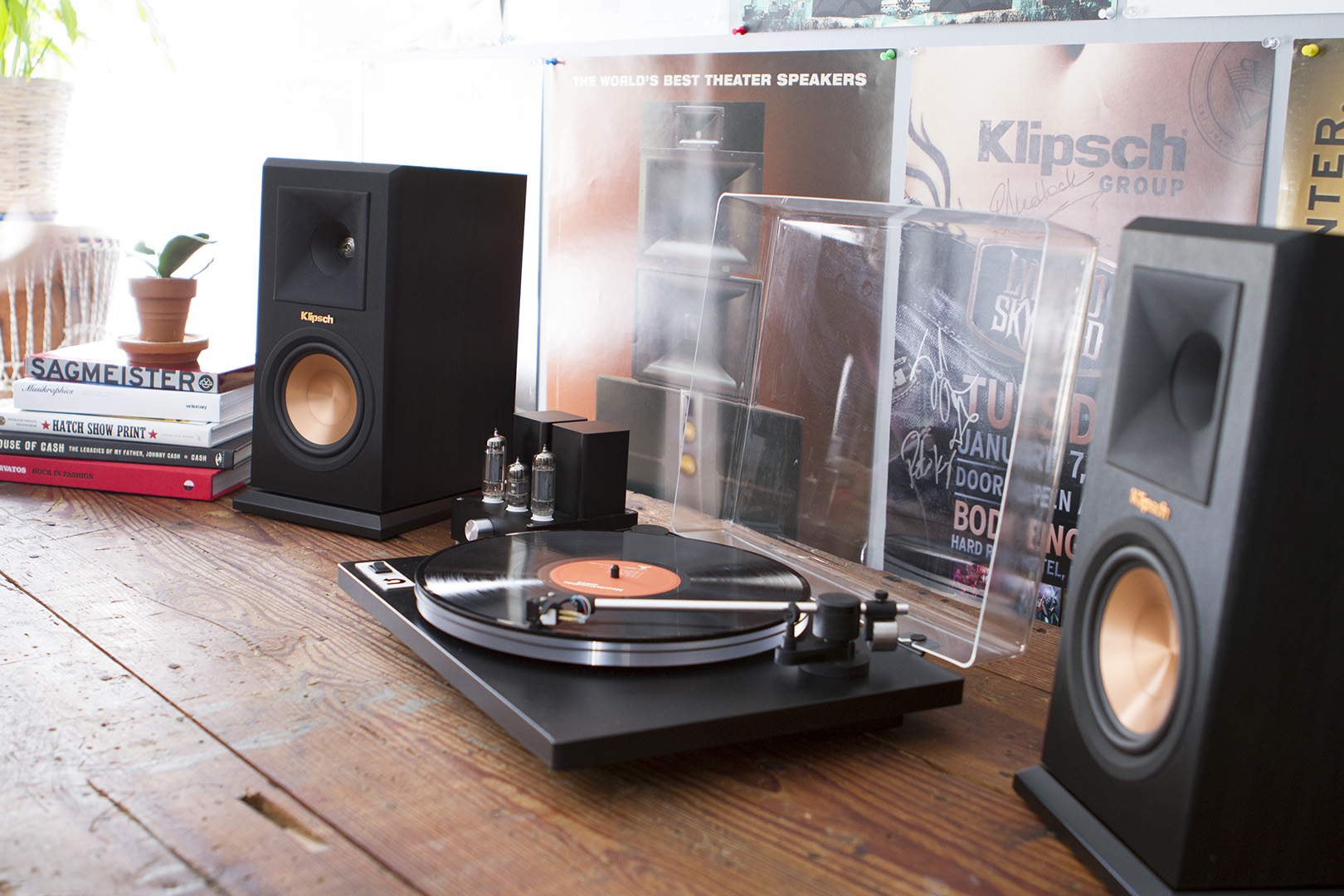The photograph captures a vibrant scene of a music setup, possibly part of an advertisement for Klipsch speakers. Positioned on a worn wooden surface, which could be either a desk or the floor, the centerpiece of the image is a sleek black record player with a clear acrylic top that is open, displaying a spinning vinyl record with an orange label. To the right and left of the turntable are high-end Klipsch speakers, recognizable by their black finish and distinctive copper-colored drivers. 

To the left of the left speaker, there's a small collection of books, with visible titles including "Sagmeister," "Hatch Show Print," and "House of Cash," topped with a terracotta pot housing a small green plant, likely an orchid. Nestled beside the turntable on the left is a compact tube amplifier, contributing to the setup's sophisticated audio equipment. 

In the background, a bulletin board is adorned with various posters. One prominently reads "The World's Best Theater Speakers," while another advertises the "Klipsch Group," and includes details of a Lynyrd Skynyrd concert on January 7th, although the year and specific details are partially obscured. This meticulously arranged scene is bathed in natural light pouring in from an unseen window, creating an inviting and nostalgic atmosphere.